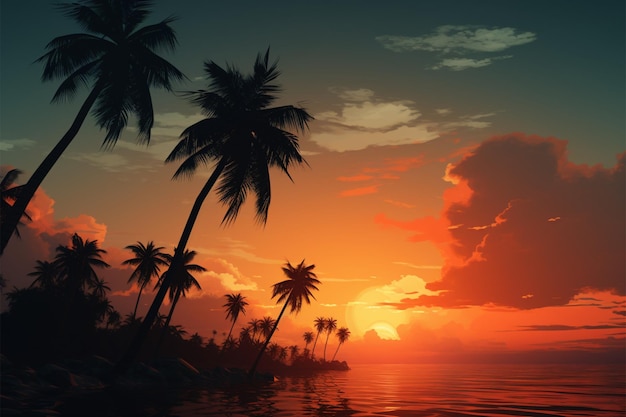This image is a stunning, computer-generated illustration of a sunset in a tropical setting, beautifully capturing the transition from day to night. The sky is a magnificent gradient of dark blue at the top, blending seamlessly into shades of pink, orange, and yellow as the sun sets behind scattered clouds. The bright yellow sun is positioned at the horizon in the center, creating a striking halo effect through the clouds. To the left of the image, the silhouettes of palm trees, both in the foreground and in the distance, lean towards the center, adding to the serene ambiance. A long peninsula full of brush and trees extends into the waterway, enhancing the tropical feel. The water on the bottom right reflects the sunset's vibrant colors, appearing as a deep burnt orange near the palm trees and transitioning to darker hues as it stretches towards the horizon. Large clouds add depth to the sky, shifting from white to red to purple as the evening approaches, making the scene both dynamic and tranquil.